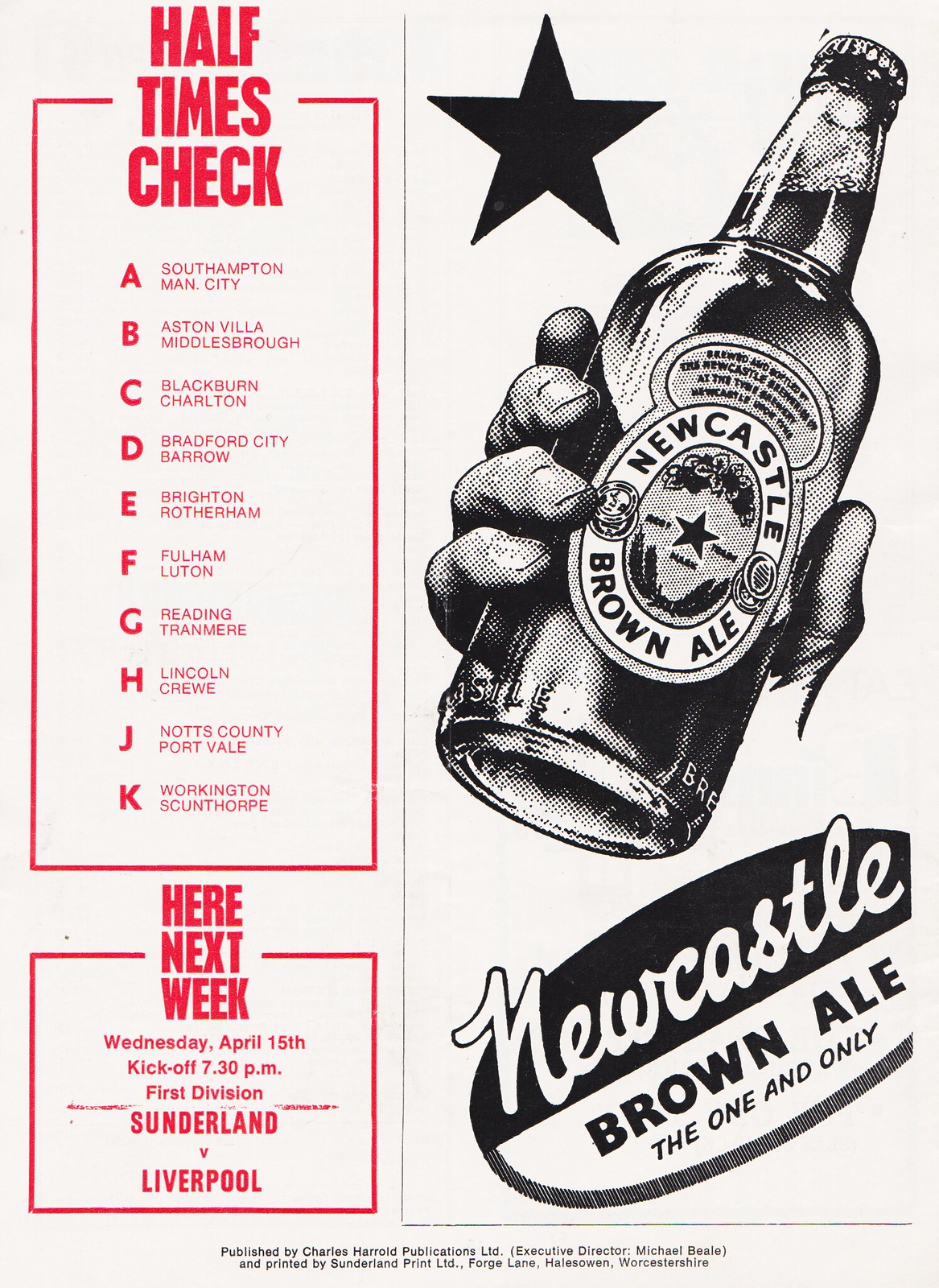The image features an advertisement with a white background showcasing Newcastle Brown Ale. On the right-hand side, there's a graphic of a hand holding a tilted beer bottle, with the label prominently displaying "Newcastle Brown Ale" in white cursive font and "the one and only" in black print, accompanied by a distinctive black star above the label and an oval-shaped label tilting slightly counterclockwise. On the left-hand side, two rectangular boxes outlined in red host a "Half Times Check" section listing letters from A to K matched with football teams such as Southampton, Man City, Blackburn, Charlton, Aston Villa, Middlesbrough, and Rotherham. Below this, the ad details an upcoming match: "Here next week, Wednesday, April 15th, kick-off 7.30pm, First Division, Sunderland vs. Liverpool." At the bottom, smaller text notes that the ad is from Worcestershire.